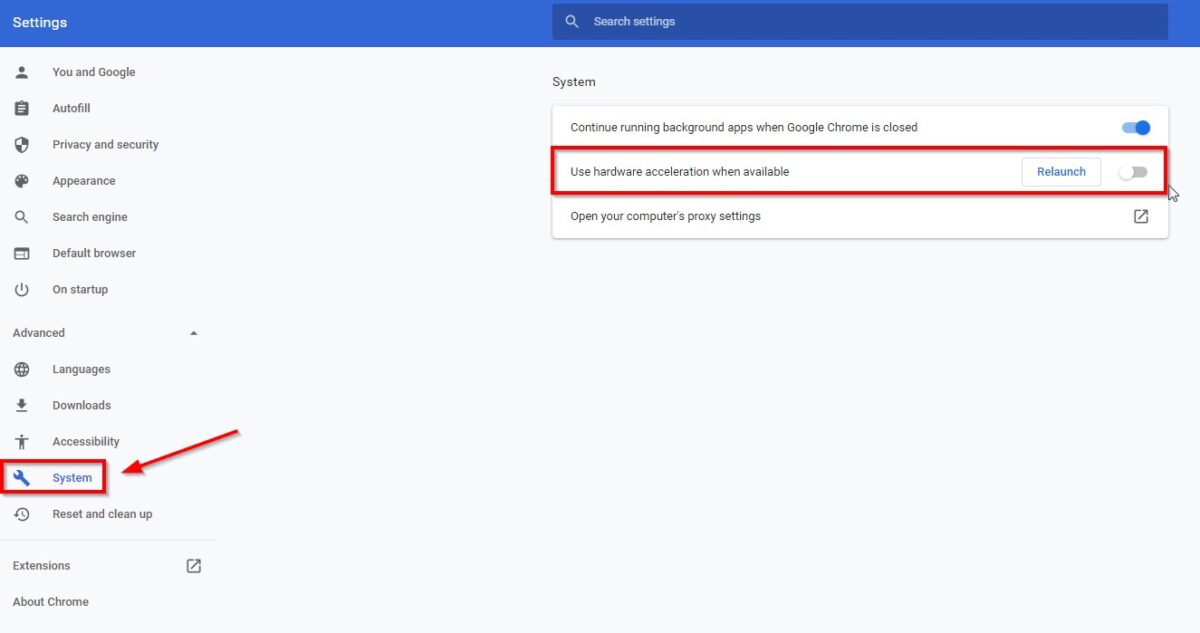Screenshot depicting the Google Chrome settings menu against a light green background. At the top, a white magnifying glass icon accompanies the text "Search settings," both in white. The settings categories listed include: You and Google, Autofill, Privacy and security, Appearance, Search engine, Default browser, On startup, Advanced, Languages, Downloads, Accessibility, and System. Each category appears in gray, while selected categories are highlighted in blue. 

A prominent red rectangle encircles the "System" category, with a red arrow pointing towards it. Inside this red rectangle, are sub-settings such as "Reset and cleanup," "Extensions," "About Chrome," and notably "System." The "Continue running background apps when Google Chrome is closed" option features a blue toggle switch set to 'on'. Below it, the "Use hardware acceleration when available" option includes a white toggle switch set to 'off' and a blue "Relaunch" button. A white cursor is positioned adjacent to the red rectangle, indicating an area of interaction.